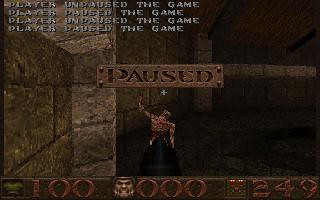This small, low-resolution color screenshot captures a paused moment in a vintage 1980s-style video game. Dominating the center of the screen is a metallic brass, bolted sign with the word "paused" displayed prominently. Below this sign, a muscular warrior, viewed from behind, stands in a dimly lit dungeon hallway, characterized by thick stone walls and intricate brickwork with visible mortar lines. The warrior, who wears a long, black skirt reaching the floor, rests his right hand against a dark stone wall, while his left arm is stretched upwards. The lower part of the image, shrouded in darkness, features a status bar displaying various attributes: an armor rating of 100, an angry face with a value of 000, and an icon that resembles a chest marked with 249. In the top-left corner, the screen repeatedly notes the player's recent actions: "player unpaused the game," "player paused the game," "player unpaused the game," and "player paused the game." The game’s primitive graphics and the atmospheric, tomb-like environment evoke a sense of nostalgia, reminiscent of early adventure and action games.